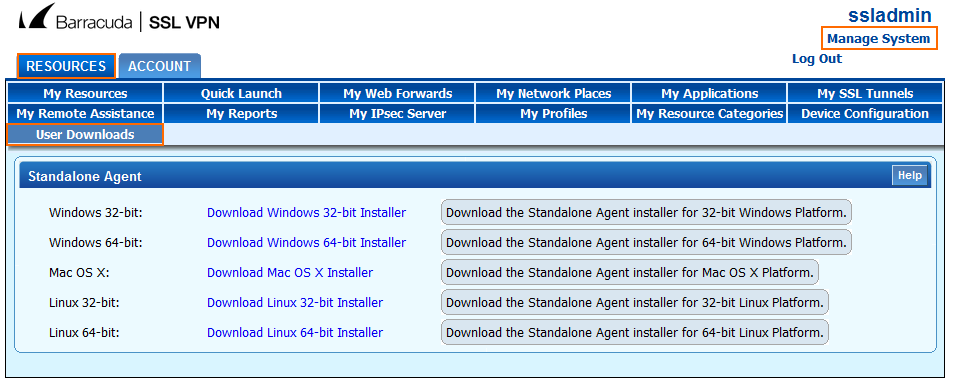A detailed screenshot of a systems management interface is displayed. The top left features a black shadow outline resembling the City Opera House, identified as 'Barracuda.' A vertical navigation menu includes options labeled 'SSL,' 'VPN,' 'SSLADMIN,' enclosed within a red border, along with 'Manage System' and 'Logout.'

The section headers are highlighted in blue, titled 'Resources' and 'Account,' followed by a sequence labeled 'Blue.' Below, various resource and management tools are listed: 'My Resources,' 'Quick Launch,' 'My Web Forwards,' 'My Network Wizard,' 'My Applications,' 'My SSL Tunnels,' 'My Role Assistants,' 'My Reports,' 'My Appcycle Server,' 'My Profiles,' 'My Resource Categories,' 'Device Configuration,' and 'User Download.'

Additionally, 'Standalone Agent' is mentioned, accompanied by text specifying operating system options: 'Windows 32-bit,' 'Windows 64-bit,' 'Mac OS X,' 'Linux 32-bit,' and 'Linux 64-bit.' Instructions include the steps to download and install the standalone agent for each platform: 'Download Windows 32-bit installer,' 'Download the Standalone Agent installer for the Windows 64-bit platform,' 'Download Mac OS X installer,' 'Download the Standalone Agent installer for the Mac OS X platform,' 'Download Linux 32-bit installer,' 'Download the Non-Standalone Agent installer for the Linux 32-bit platform,' 'Download Linux 64-bit installer,' and 'Download the Standalone Agent installer for the Linux 64-bit Lithium platform.'